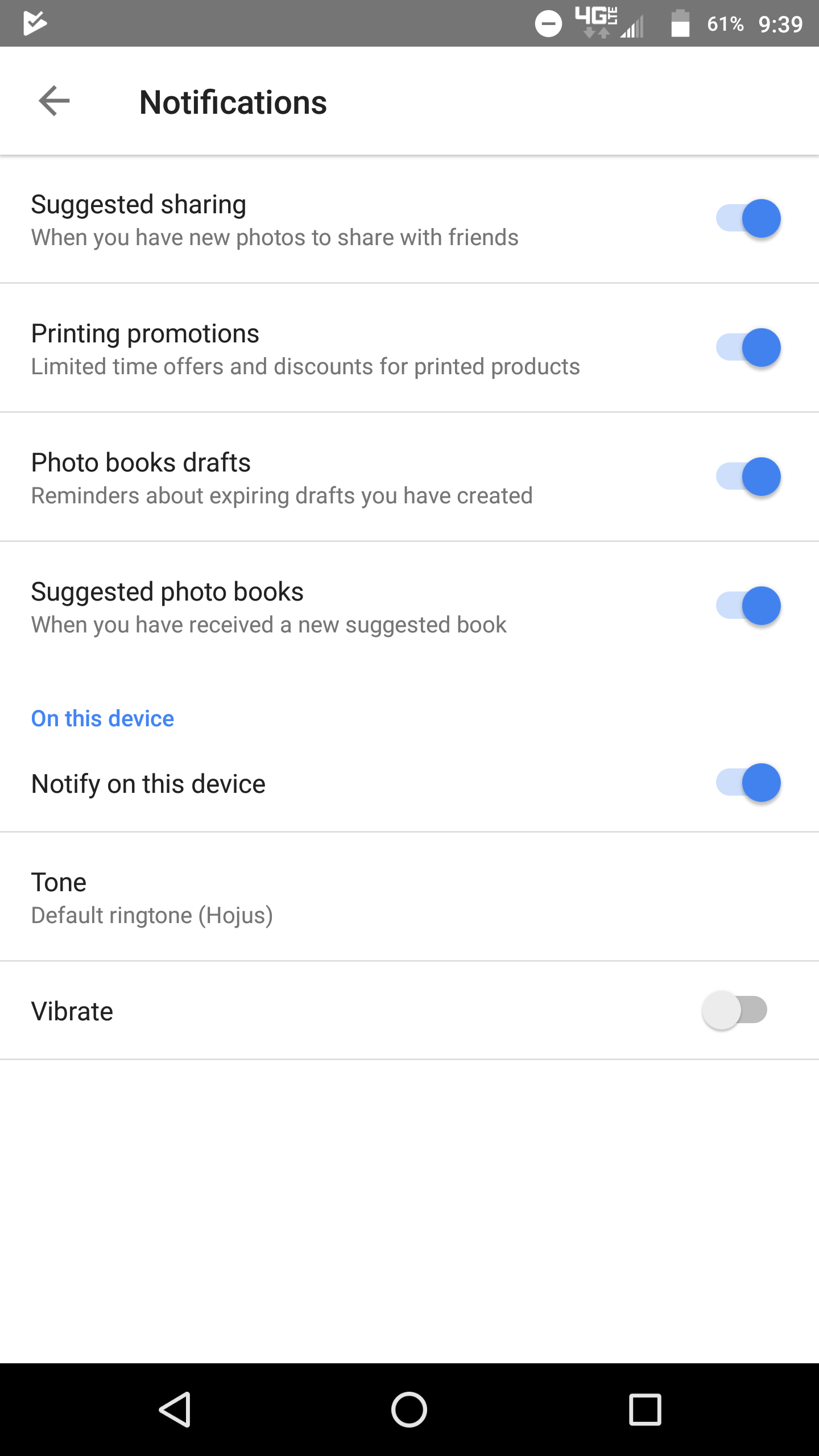The image captures a screenshot from a cell phone's notification settings page. At the top, the status bar displays a "4G LTE" network connection, a battery level at 61%, and a timestamp of 9:39. Below the status bar, the screen is titled "Notifications" in bold.

The notifications are listed as follows, each with its current setting:

1. **Suggested Sharing**: Notifies the user when there are new photos to share with friends. This notification is enabled.
   
2. **Printing Promotions**: Informs the user about limited-time offers and discounts for printed products. This notification is enabled.
   
3. **Photo Book Drafts**: Reminds the user about expiring drafts they have created. This notification is enabled.
   
4. **Suggested Photo Books**: Alerts the user when a new suggested photo book is available. This notification is enabled. Below this, there is a clickable link titled "On this device" in blue.
   
5. **Notify on this device**: This notification is enabled.

Below the notification settings, there is a section for sound settings:

6. **Tone**: Displays the current default ringtone, "H-O-J-U-S", but does not provide an option to toggle this notification on or off.
   
7. **Vibrate**: The vibration setting is currently turned off.

Each notification setting is clearly demarcated, providing a comprehensive overview of the notification preferences on the device.